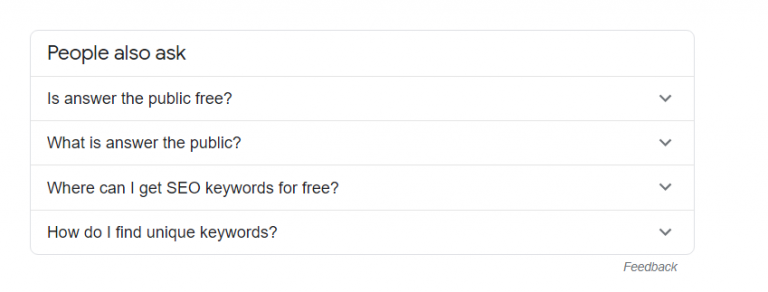This image is a screenshot of a web page section titled "People also ask," featuring a list of frequently queried questions. Each question is accompanied by a drop-down arrow that hints at additional information available upon expansion. The questions listed are: "Is Answer the Public free?", "What is Answer the Public?", "Where can I get SEO keywords for free?", and "How do I find unique keywords?". Below these inquiries, a "Feedback" option is available at the bottom right corner of the section. Separating each question is a thin gray horizontal line. The entire text is printed in black, and the image is devoid of any illustrative, photographic, or graphic elements. There are no depictions of people, animals, plants, buildings, or any other objects, making it a purely textual representation.